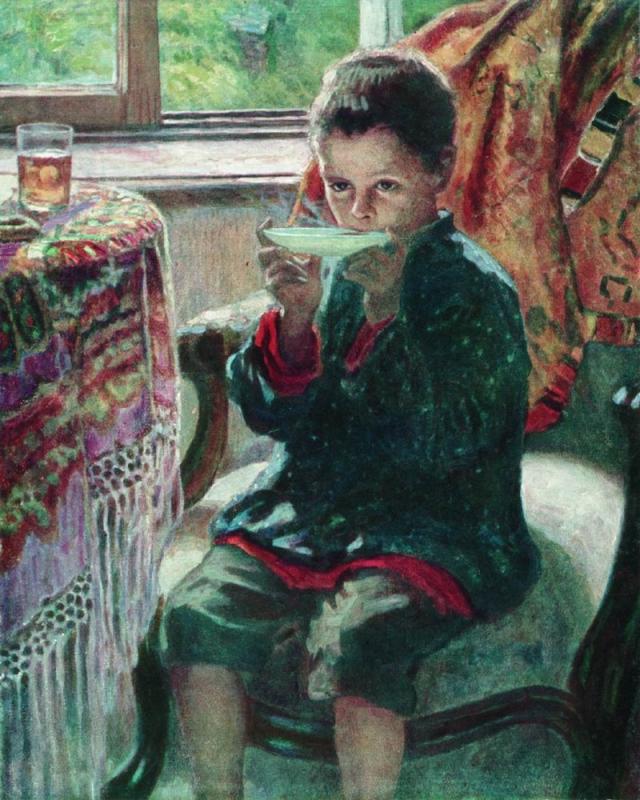In this detailed painting, a young boy, around eight or nine years old, is depicted sitting on an ornate armchair draped with an ornamental blanket that features red and yellow hues. The boy is dressed in a green jacket adorned with tiny white specks over a red undershirt. His green capri pants expose his calves but not his feet. With short brown hair, he appears to be concentrating as he sips from a shallow bowl or saucer held up to his mouth. Beside him, to the left, there is a table covered with a colorful tablecloth decorated in shades of purple, pink, red, green, and white fringes. On the table sits a clear glass of iced tea and another indistinguishable small object. Behind him is the bottom third of a window, through which greenery outside can be faintly seen. The scene, likely set in a living room or kitchen, is rendered in a style that merges photographic realism with painterly elements.